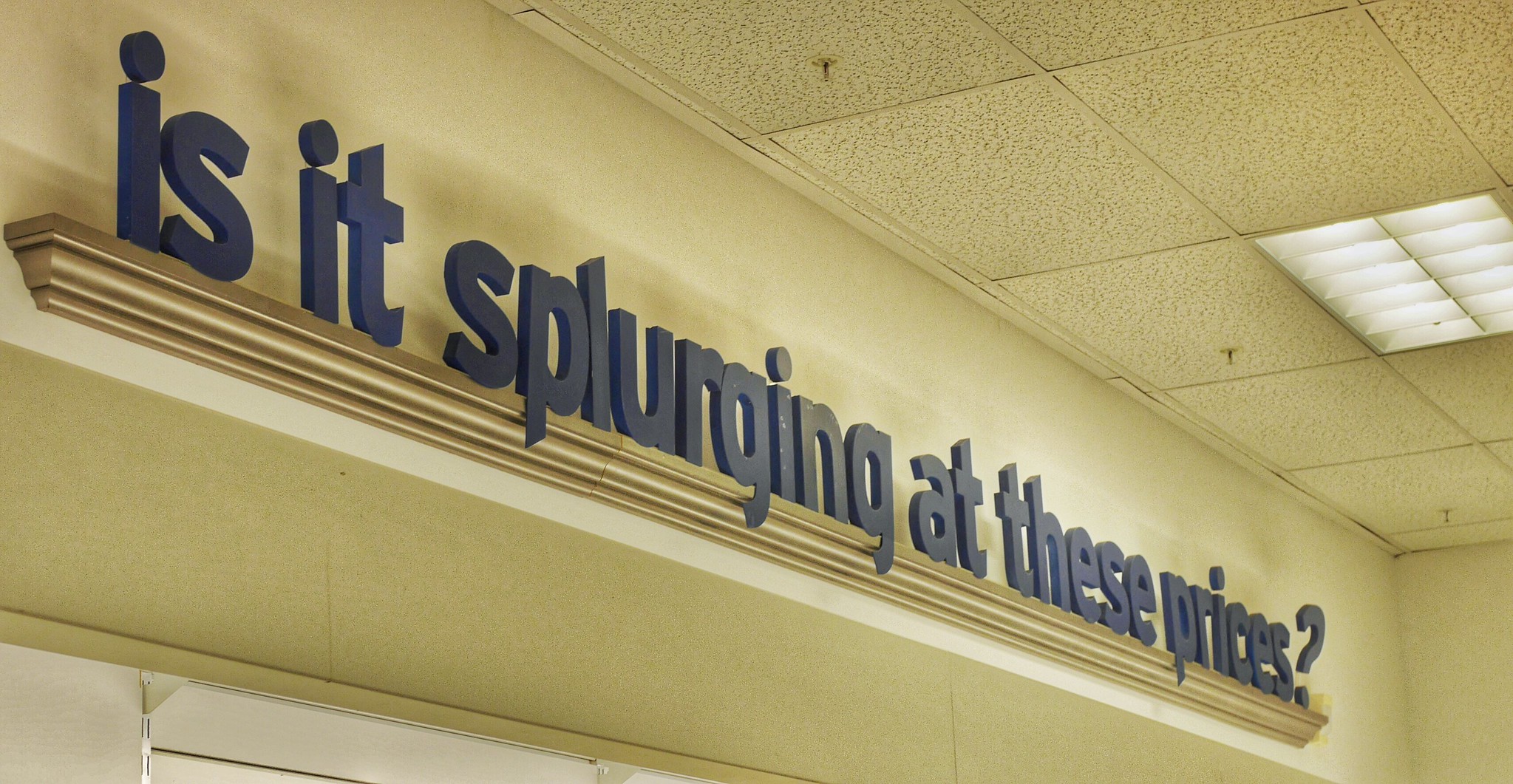The image captures the interior of an older building, focusing on the ceiling and upper part of the wall. The ceiling consists of drop tiles with a grid pattern of large squares, interspersed with fire sprinklers and a fluorescent light fixture on the right side, and exhibits signs of age with dingy, stained yellow tiles and some brownish-black spots. In the upper right corner, there is also a vent. Below the ceiling, an off-white or beige wall is visible. Dominating the wall is a long, rectangular gold shelf supporting tall, blue, 3D letters, approximately six to eight inches in height, spelling out the phrase, "Is it splurging at these prices?". The shelf and letters take up a significant portion of the image, and the setting appears to be a business establishment, likely indoors.